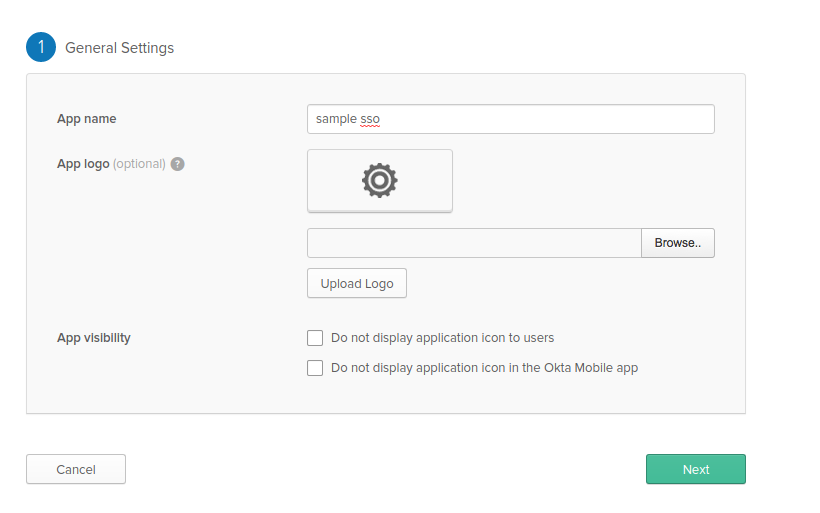The image depicts a square-shaped webpage with a minimalistic design featuring gray and light blue colors. At the top of the page, a blue circle with the number "1" is positioned next to the bold text "General Settings." The upper-left corner displays the app name, "Sample SSO".

Below the heading, the page includes fields labeled for "App Name" and "App Logo (Optional)," accompanied by a question mark icon for additional information and a settings gear icon. The central area of the page provides a section to upload a logo, with a prompt to "Browse" for the file once clicked.

The lower portion of the page offers options under "App Visibility," allowing users to select either "Do not display application icons to users" or "Do not display application icon in the Okta mobile app." Finally, at the bottom of the page, there are two buttons: "Cancel" and "Next."

The page has a simple and uncluttered interface, predominantly using grayed-out and white colors. Key options and labels are highlighted in bold to emphasize their importance. Overall, the design maintains a clean aesthetic with a focus on usability and essential settings.